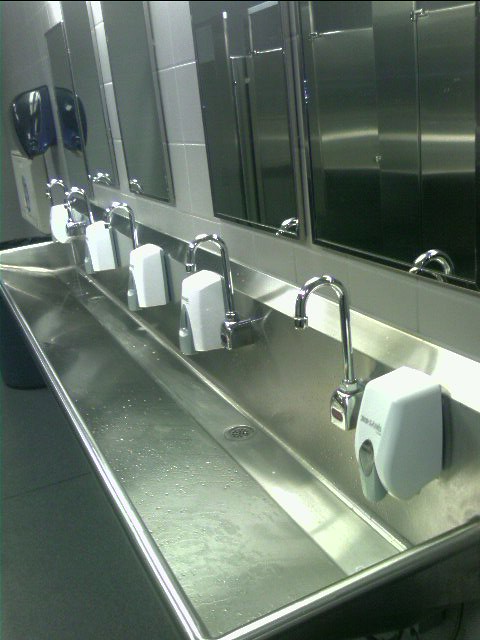The image depicts a commercial bathroom with a long, wall-mounted metal sink featuring five U-shaped faucets evenly spaced along its length. Each faucet is accompanied by a white soap dispenser with a gray push handle. The sink has a gently sloping surface that channels water towards two central drains. Above each soap dispenser is a tall, rectangular mirror. In the background, a blackish-blue paper towel dispenser is mounted on the wall above a large trash can. To the right of the paper towel dispenser is a wall-mounted baby-changing station that can be folded down for use. The bathroom floor is gray, and scattered water droplets can be seen in the sink, indicating its recent use. There are no people present in the image.